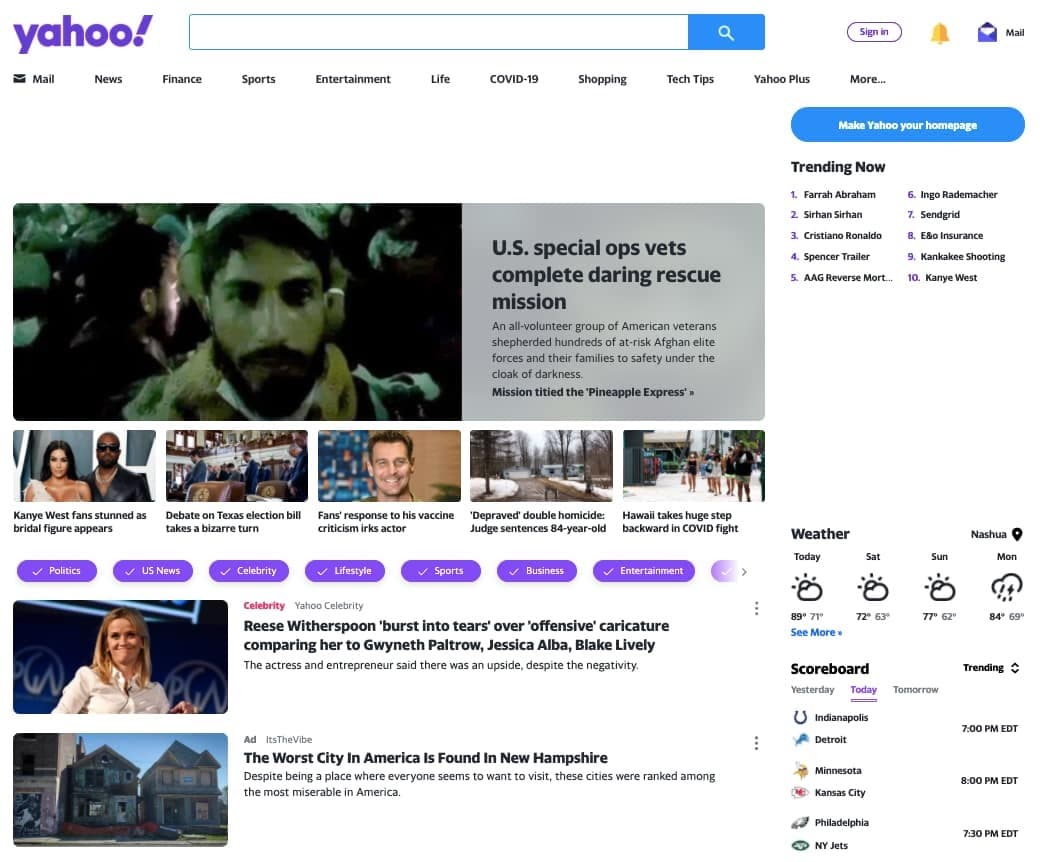The image depicts a webpage with a predominantly white background, making the edges nearly indistinguishable. At the top of the page is the Yahoo logo situated in the upper left corner. Adjacent to it is a search bar, accompanied by a blue search button featuring a magnifying glass icon. Further to the right is a purple-outlined button labeled "Sign In" in purple text. Next to this is a notifications icon, represented by a gold bell, followed by an open blue envelope icon with the word "Mail" in black text beside it.

Beneath these elements is a horizontal menu bar offering various categories: Mail, News, Finance, Sports, Entertainment, Life, COVID-19, Shopping, Tech Tips, Yahoo Plus, and More.

Below this menu, the left-hand side prominently displays a headline article, featuring an image of a man likely in his 30s, with a full beard, standing in a crowd under dim lighting. To the right of the image, a gray text box contains the article's title: "US Special Ops Vets Complete Daring Rescue Mission," followed by a brief paragraph. Below this headline, there are seven additional articles listed.